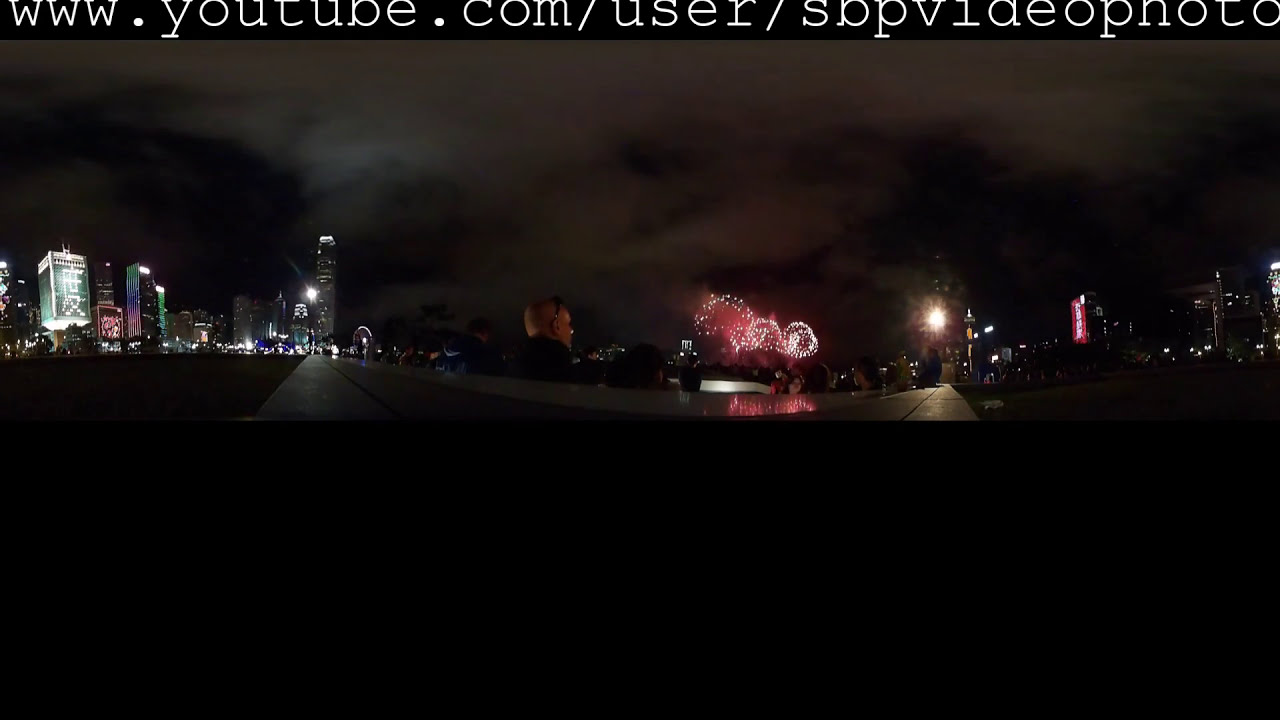The image is a nighttime, 360-degree panoramic shot of a metropolitan area with a heavily clouded sky illuminated by light pollution. Centered in the photo, vibrant fireworks with red smoke and white sparkles burst and cascade over the city’s skyline. On the left, a collection of high-rise buildings stand prominently, glowing in green, red, and blue lights. To the right, a significant red sign with white writing is noticeable among other illuminated structures. The lower half of the image is obscured by a black bar, while the top features the text "www.youtube.com/user/SBPVideoPhotos" in white font. Although the scene is dark and somewhat foreboding, it is bustling with activity, capturing the essence of a festive city night, possibly during a fireworks display.